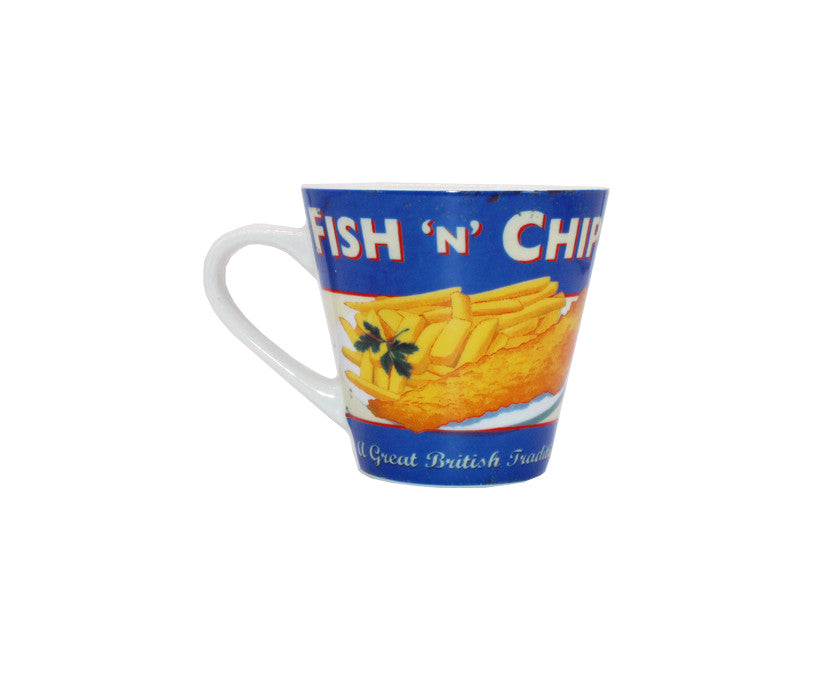The image depicts a small coffee mug with a white handle situated on the left side. The mug's overall color scheme includes a blue exterior and a white interior. The design features a blue background with white text outlined in red that reads "Fish 'n' Chips." Below this text, a detailed image of a classic fish and chips dish is displayed on a white and red plate, complete with a piece of fried, battered fish alongside french fries, accentuated by a small sprig of green parsley as garnish. Additionally, at the bottom of the mug, in white cursive text on a blue banner, the phrase "A Great British Tradition" is inscribed, reflecting the nostalgic and traditional theme of the design. The mug is set against a clean, white background, providing a stark contrast that highlights the intricate details and colors of the mug's artwork.